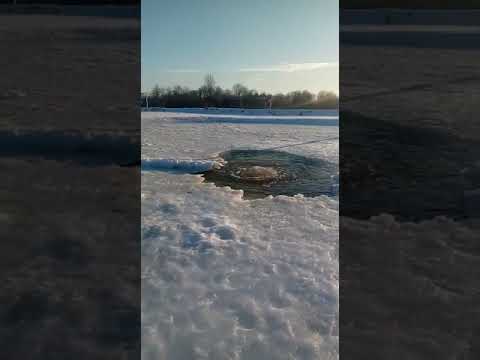In this photograph, a frozen lake is captured during the daytime, with a thick sheet of ice covering the surface. Prominent borders on the left and right sides, which consist of the enhanced and darkened edges of the original image, frame the main picture. At the center of the lake, a hole has been broken through the ice, revealing bubbling water and a dark brown mass, possibly suggesting the presence of fish. The scene is somewhat blurry, adding ambiguity to whether a fishing line or shadow streaks into or out of the hole.

The ice across the lake is mostly white, with hints of blue that might be reflections of the sky. Towards the horizon, shadows stretch across the lake, and in the distance, the landscape gently inclines, with snow-covered hills dotted with trees. Among these, some trees are bare, while others retain foliage. Above, the sky is a pale blue, lightly decorated with wisps of white clouds. This picturesque and serene setting is captured in a detailed and textured photograph that conveys the stillness and ever-present life just beneath the icy surface.